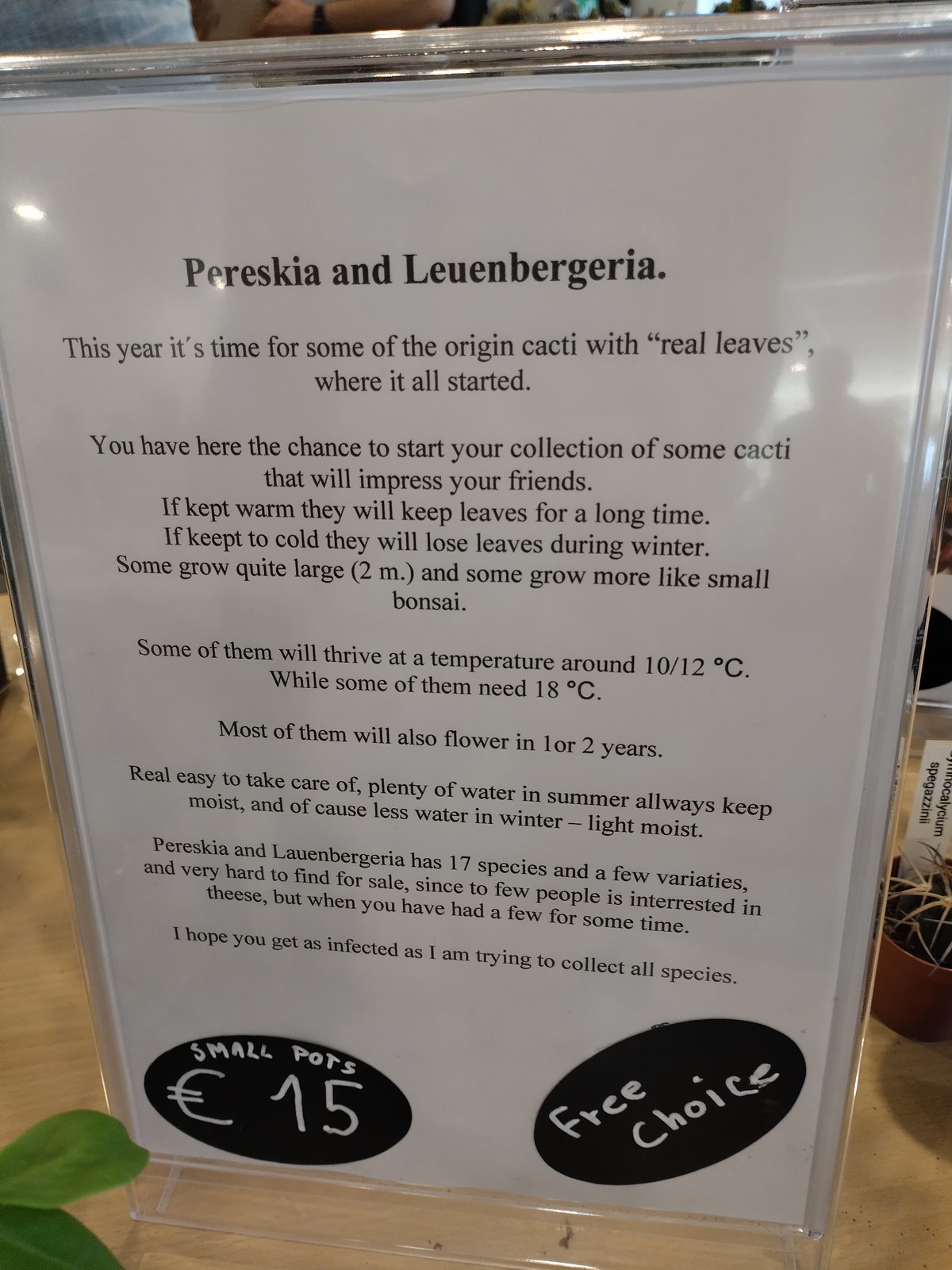Displayed on a glossy light brown wooden table, this laminated white paper stands upright in a clear plastic holder. The detailed menu, titled in bold black lettering, spells out "Pereskia and Luenbergeria." It promotes a selection of origin cacti noted for their real leaves, highlighting their impressive and diverse nature. At the bottom left and corner edges, two green leaves and a spiky plant add a touch of visual appeal.

The menu explains that these cacti, with 17 distinct species, offer a unique opportunity to start a collection that will captivate friends. It details the care requirements: they retain leaves longer when kept warm but may lose them in winter if too cold. Optimal growth temperatures range from 10-12°C for some species to 18°C for others, with potential flowering in one to two years. Additionally, growth variations are noted, from small bonsai-like sizes to larger plants reaching up to 2 meters.

At the bottom left corner of the menu, within a black oval, it mentions the availability of small pots priced at 15 Euros, with another circle indicating a "free choice." Finally, it advises consistent watering in summer to keep the soil moist, tapering off in winter to a light mist. The beige color of the table subtly complements the overall display.